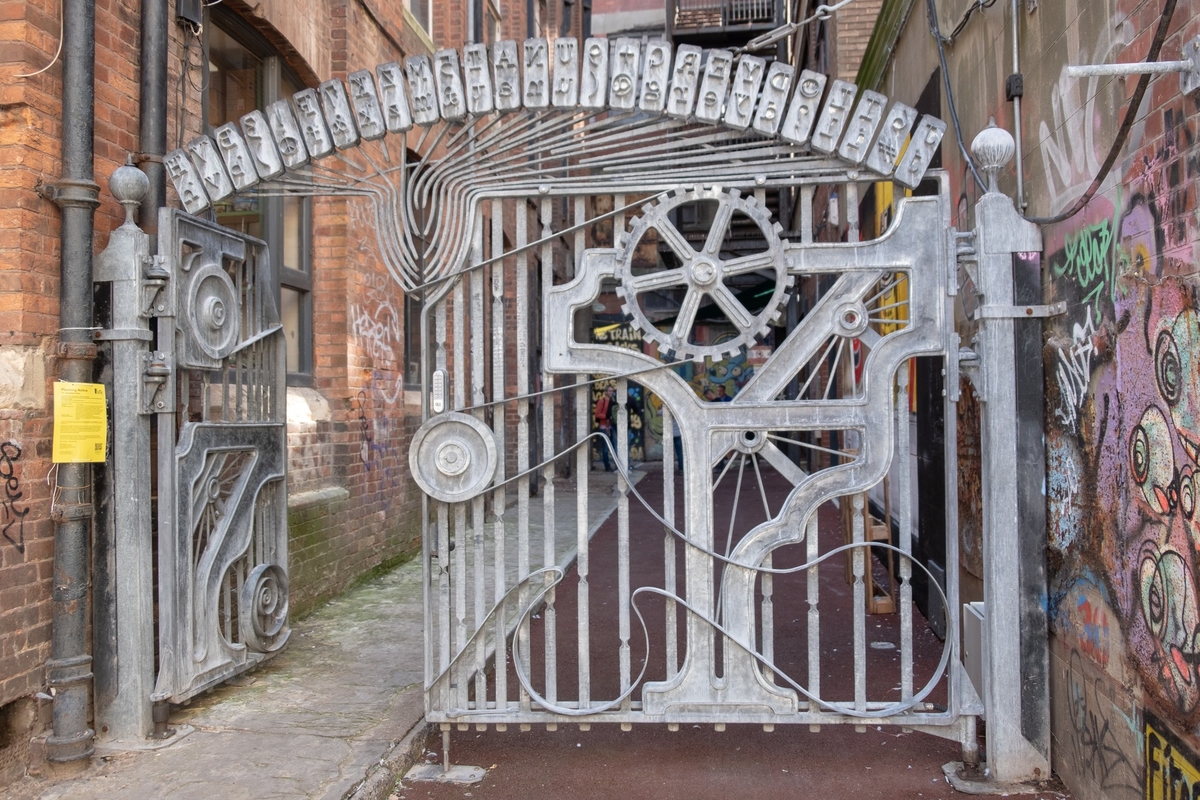The photograph features a detailed, intricate gate centered between two brick buildings. The gate, constructed from gray wrought iron, has an elaborate design that mimics the look of various cogs and interconnected bars, with some cogs appearing damaged or missing. This silver-gray gate includes an overhanging arch adorned with vertical rectangles, some bearing indistinct letters like "K" and "W." The gate is set on large square posts topped with ornamental balls, leading to an alleyway with a tan pathway on the right and a raised gray concrete slab sidewalk on the left, covered in green moss and vegetation. The brick building on the right showcases graffiti and street art, while the building on the left is primarily a reddish-orange color with hints of graffiti. Additionally, a yellow notice is attached to a pole on one of the buildings. The gate itself has one door open, inviting viewers to see beyond into the alley.